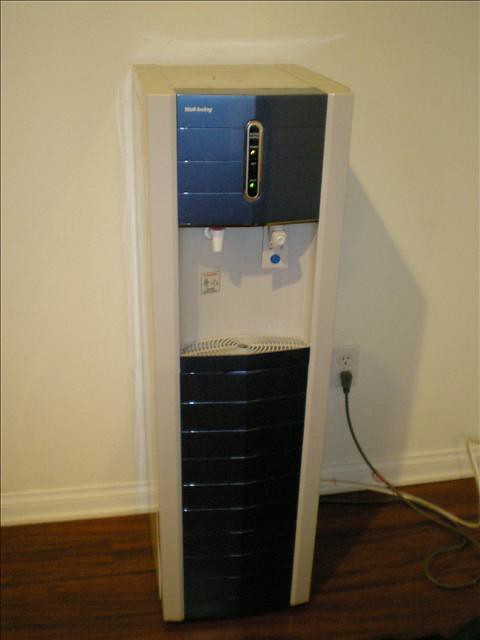The image showcases a tall, rectangular, white plastic water dispenser positioned against a white painted wall and set on a dark brown, likely wooden, floor. The water dispenser features a central dark navy blue, metallic-looking panel with shiny horizontal ridges, which divides the otherwise white exterior. At the top of this panel, there's a control area with two indicator lights and some writing. 

In the middle of the dispenser are two nozzles: the left one, likely for hot water, has a red top portion and a nearby warning sign indicating hot water, while the right one, presumably for cold water, has something hanging from it—a white tag with a blue circle. Directly below the nozzles is a tray with horizontal ridges for drainage when a cup or bottle is placed underneath to fill up. 

The dispenser is plugged into a beige US outlet on the right side, with its cable and plug extending down to the floor. Due to the lighting from the top left corner, the shadow of the water dispenser extends towards the bottom right.